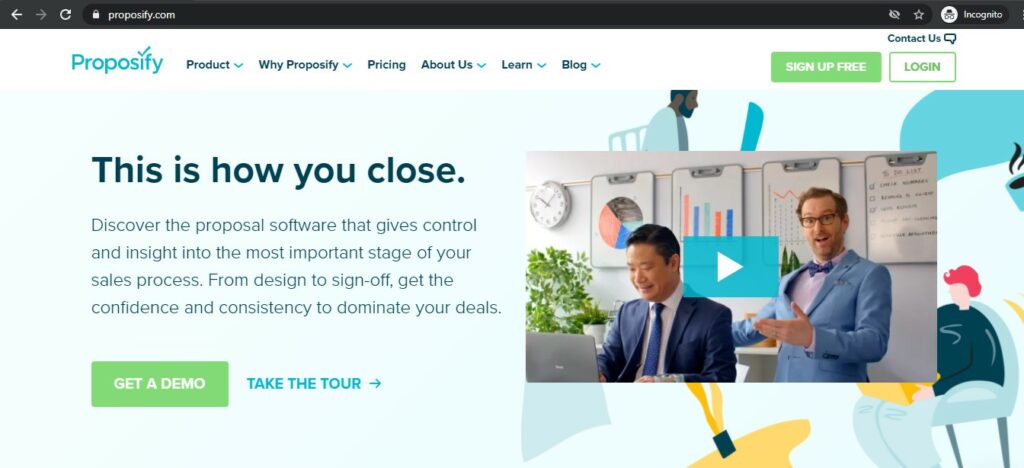This image is a screenshot taken from the Proposify website. At the top of the screenshot, there is a black rectangular box displaying the text "Proposify" and its URL, "proposify.com." The interface includes navigation buttons such as a back button and a refresh button in the top right corner, along with an incognito icon and three other icons.

Below this, a menu bar contains options in black text: "Product," "Why Proposify," "Pricing," "About Us," "Learn," and "Blog." The active section, highlighted in teal, can be clicked to explore further.

Underneath the menu, there is a prominent section with a headline that reads, "This is how you close." The accompanying text explains the benefits of the proposal software, stating, "Discover the proposal software that gives control and insight into the most important stage of your sales process from design to sign off. Get the confidence and consistency to dominate your deals."

To the right of this paragraph, there is a video thumbnail featuring two men in professional attire. One man is wearing a blue bow tie and a matching blue suit coat. Both men are smiling, creating an inviting preview for the video. There are options to either watch the video directly or proceed with a demo by clicking on a green button labeled "Get a Demo." Alternatively, users can choose to explore further by clicking on a blue button labeled "Take the Tour."